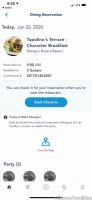In this blurry screenshot, set against a light gray background, the upper left corner features some text that is indistinguishable, possibly numbers or words. The upper right corner shows a clearly visible battery icon indicating a full charge. Centered in the middle of the image, in black text, the words "dining reservation" are somewhat discernible. Directly below this, in bold black text, the text appears to read "Today, January 22nd, 2020," indicating the date of the reservation. Although the restaurant's name remains unclear, there is a circular image that likely depicts the restaurant's interior. Below this image is a blue action button with white text, the content of which is unreadable. At the bottom of the screenshot, the text "party three" is legible, indicating the number of people for the dining reservation.